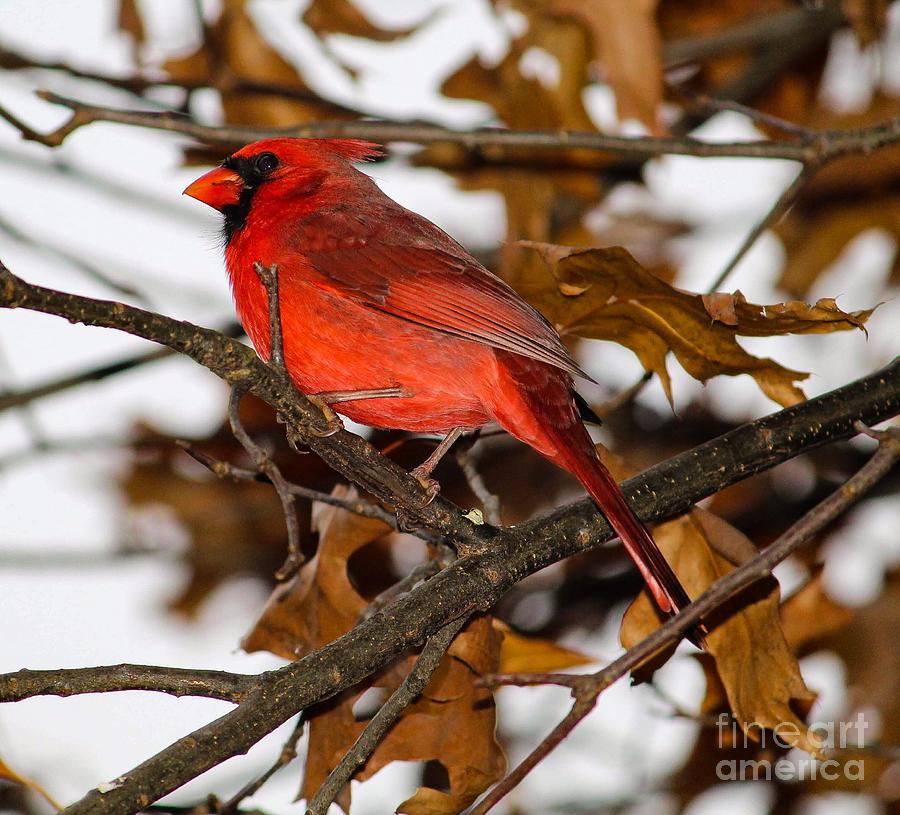This photograph showcases a striking cardinal perched gracefully on a dark brown oak tree branch in the wilderness. The bird, predominantly a beautiful shade of red, features distinct black markings around its eyes and beak, which is an orange-red hue. Its long tail feather and folded wings contribute to its full-bodied, vibrant appearance. The side view captures the cardinal looking to the left, with its tiny claws firmly clutching the branch. Surrounding the bird are dried, crinkly oak leaves, contributing to the autumnal feel of the scene. The background is an ethereal white, possibly indicative of snow, adding a serene touch. The image is bathed in sunlight, further illuminating the cardinal's radiant plumage. At the bottom right, a watermark reads "Fine Art America," suggesting the source of this exquisite nature photograph.